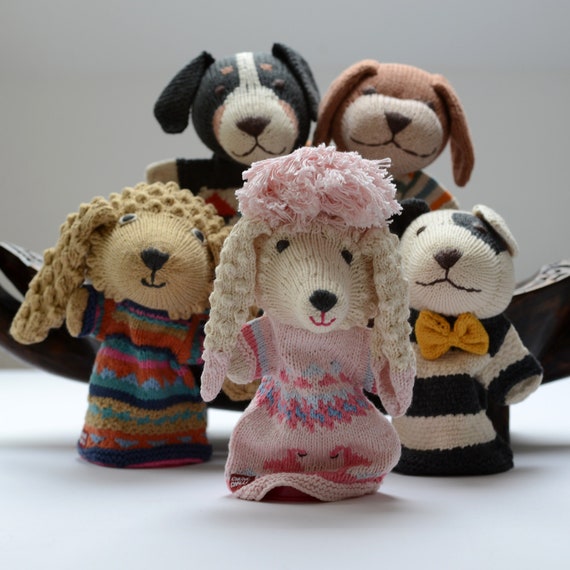The image features five handcrafted, crochet dog puppets positioned in front of a plain white background. Prominently in the center is a white poodle adorned with a pink flower in her hair, wearing a pink dress decorated with pink flamingos. She has black eyes, a black nose, and a subtle smile. On the left, there's a brown dog with googly eyes, sporting a sweater with blue, pink, orange, red, and brown patches, and featuring long black ears. To her left stands another brown dog with fluffy ears, dressed in a multicolored sweater. On the right, a Dalmatian-like dog, white with a large black patch over one eye, wears a black-and-white striped sweater paired with an orange bow tie. Behind these three, on the right, is a simple brown dog with a white muzzle, also in a striped shirt, while on the left, partially hidden, another dark-colored dog with white and brown patches peeks out. Each puppet appears to be meticulously made, reminiscent of sewn-together old socks or blankets, enhancing their charming, handmade appeal.